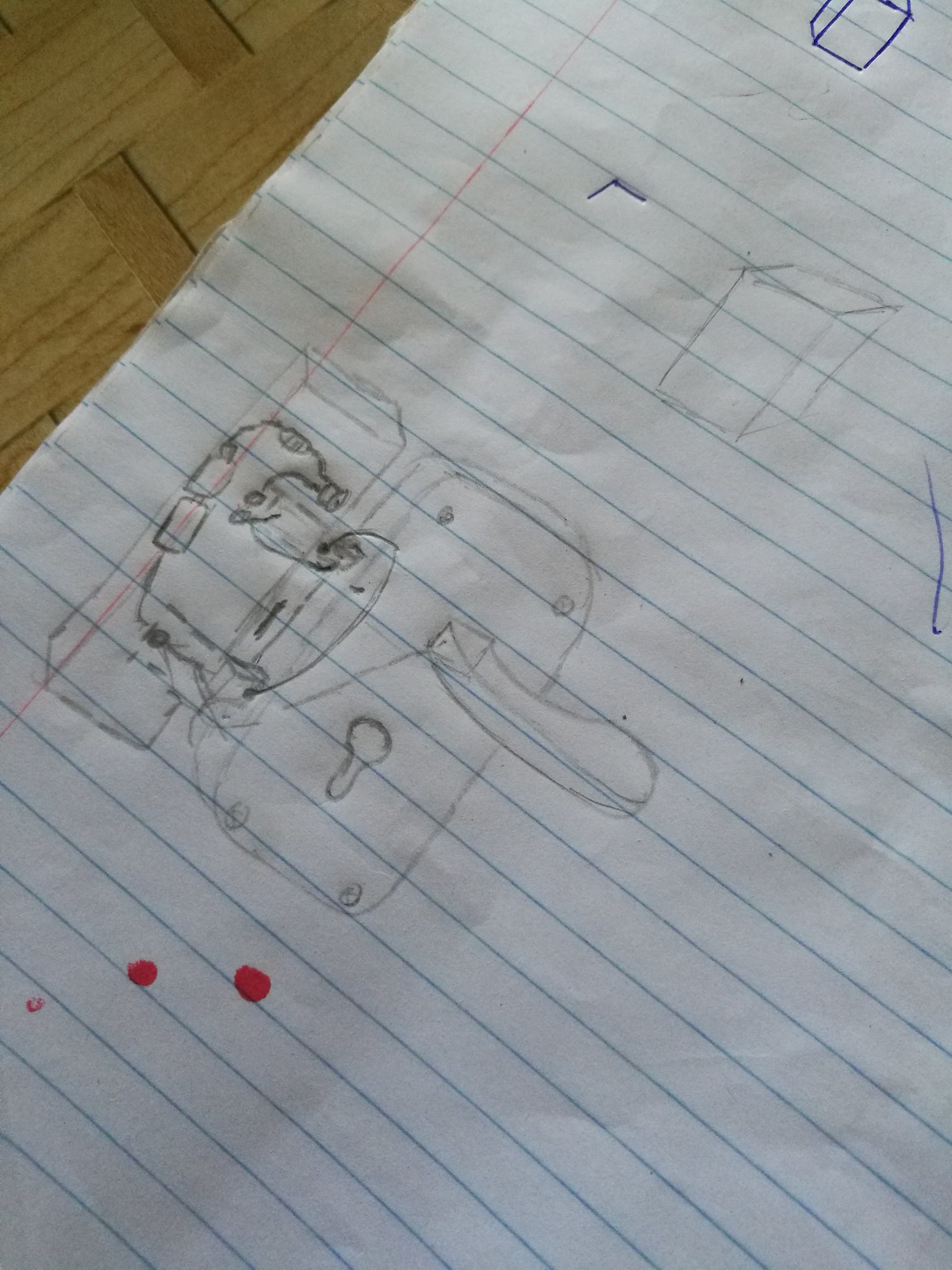A wrinkled piece of lined paper, suggesting it has been carried around, is partially visible on a tabletop. The paper features a drawing. At the top of the visible drawing, there is a 3D-like box with a stray blue line adjacent to it. Below that, there is a rectangle with two solid circles at the top, resembling a handle and a keyhole. To the right of this rectangle is another rectangular shape with indistinguishable elements.